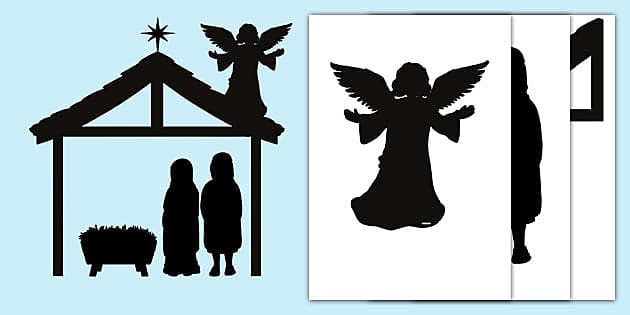The image depicts an intricate nativity silhouette scene set against a greenish-gray background. To the left, a detailed stable features an angel perched on the roof, with a star atop the peak. Below the roof, two figures, presumably Mary and Joseph, stand beside a manger filled with hay. The stable is supported by two vertical beams on either side, creating a clear and distinct frame. On the right side of the image, three overlapping white cards showcase individual black silhouettes. The top card prominently features an angel with outstretched wings and flowing robes. This card partially covers the middle card, which shows the silhouette of a standing figure. The bottom card is mostly obscured, revealing only a portion of the stable roof within a black frame. The entire composition captures the essence of a nativity scene, with emphasis on the angelic figure and the stable's simple yet evocative structure.